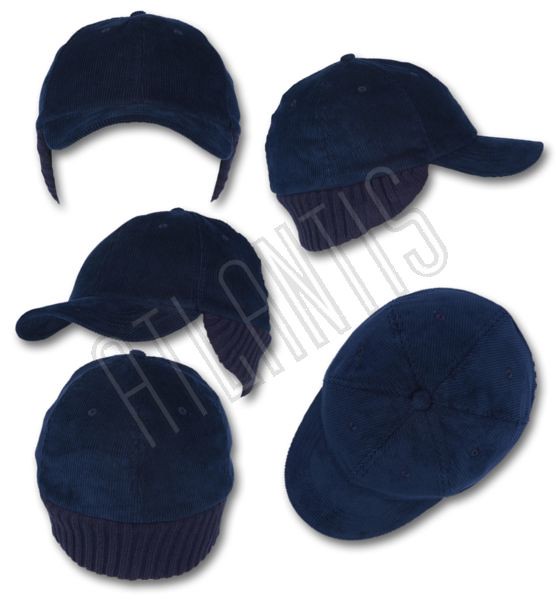This color photograph showcases five dark blue winter ball caps arranged on a white surface. Each cap is depicted from a different angle: one from the front, two side profiles (left and right), one from the back, and one from the top, allowing for a comprehensive view of the design. The caps, which feature a small button at the top where the six sections of the cap converge, have ear flaps made of material similar to that of a ski cap, extending to cover the ears and back of the head when worn. A faint, diagonal watermark spans the center of the image, spelling out "Atlantis" in capital letters, indicating the brand of these stylish caps.